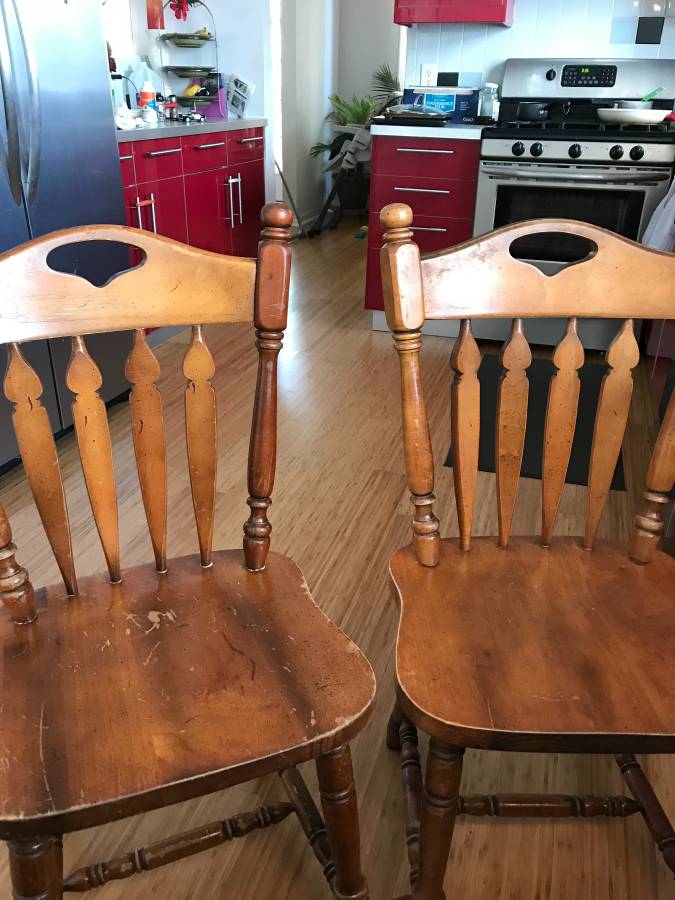This photograph captures a nostalgic kitchen setting, dominated by two classic wooden kitchen chairs, placed in the foreground on a light hardwood floor. These chairs, with their thin wooden legs and distinctive rounded seats, feature an oval cut-out in the top brace and decorative wooden spindles on the backrest. The chairs are reminiscent of a style commonly seen in American homes from years past, marked by their sturdy oak construction and slightly scratched surfaces.

In the background, the kitchen is characterized by its red cabinetry with silver handles, adding a vibrant touch contrasted by the white countertops. Prominently, there is a white stove with a matching oven and a black top, beside a small red cabinet section with four drawers and a single upper cabinet. Adjacent to these elements, a silver refrigerator stands to the left, completing the appliance trio. The kitchen sink, positioned towards the left side, complements the setup, enhancing the practical and welcoming atmosphere of this homey kitchen space. Subtle details like green plants atop the cabinetry add a fresh, lively element to the scene.